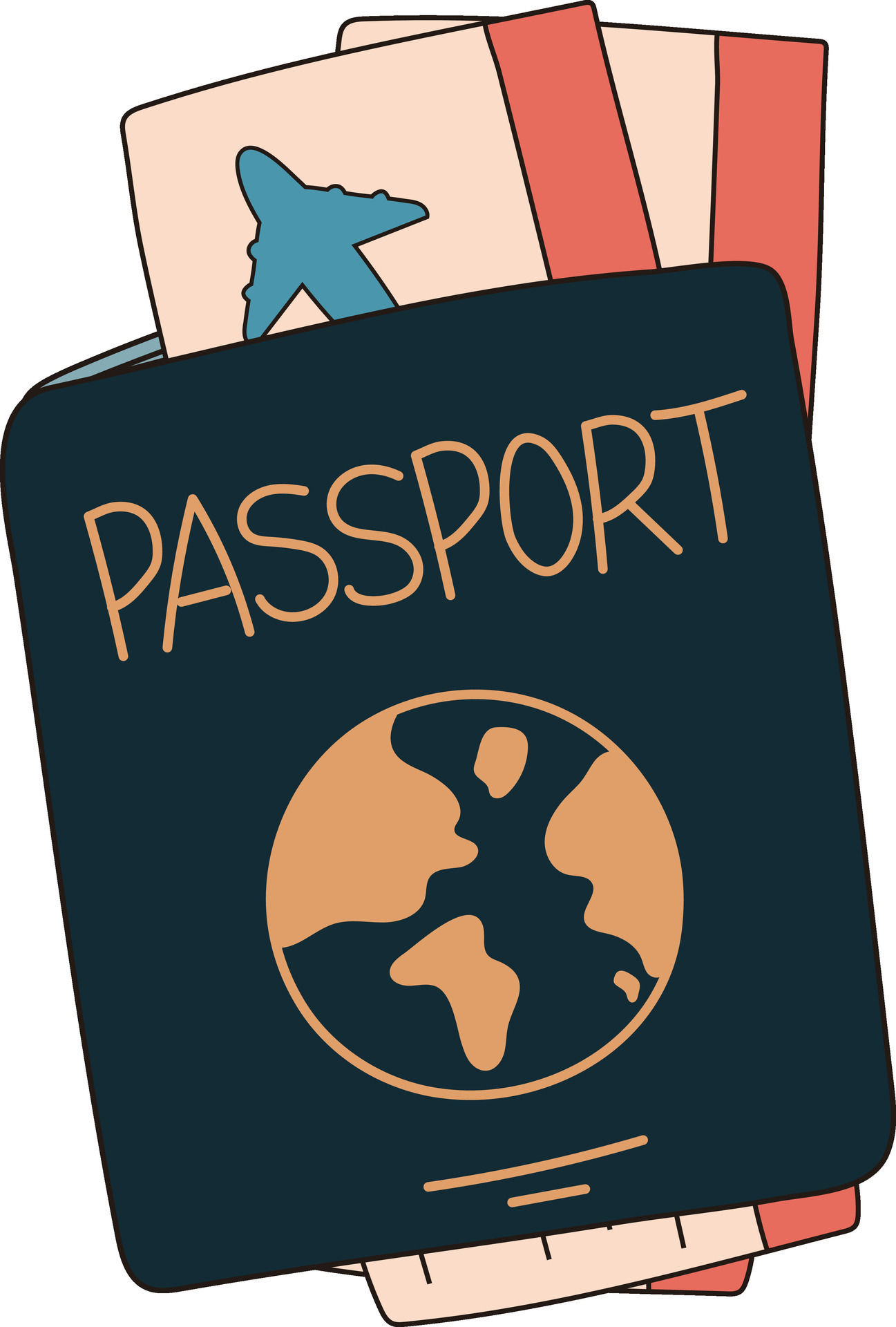This image is a cartoony, colored drawing of a slightly tilted dark blue passport. On the cover of the passport, the word "PASSPORT" is prominently featured at the top in large, capitalized, yellow letters. Below this, there is a drawing of the Earth positioned just beneath the middle. Further down, there are two horizontal yellow lines, with the top line being longer than the one below it. 

Emerging from the top of the passport are the ends of two airline tickets. The left ticket features a pink section with a blue plane drawn on it and a red border on the right side. This ticket extends down behind the passport cover. To the right of this, another similarly colored ticket (pink with a red border) is slightly visible, also descending into the passport. 

At the bottom of the passport, the ends of these tickets reappear; slight hints of pink and red from the ticket edges can be seen protruding. The drawing, while not highly detailed or lifelike, effectively conveys that the passport contains two airline tickets, recognizable by the identifiable albeit crudely drawn airplane on the top ticket.